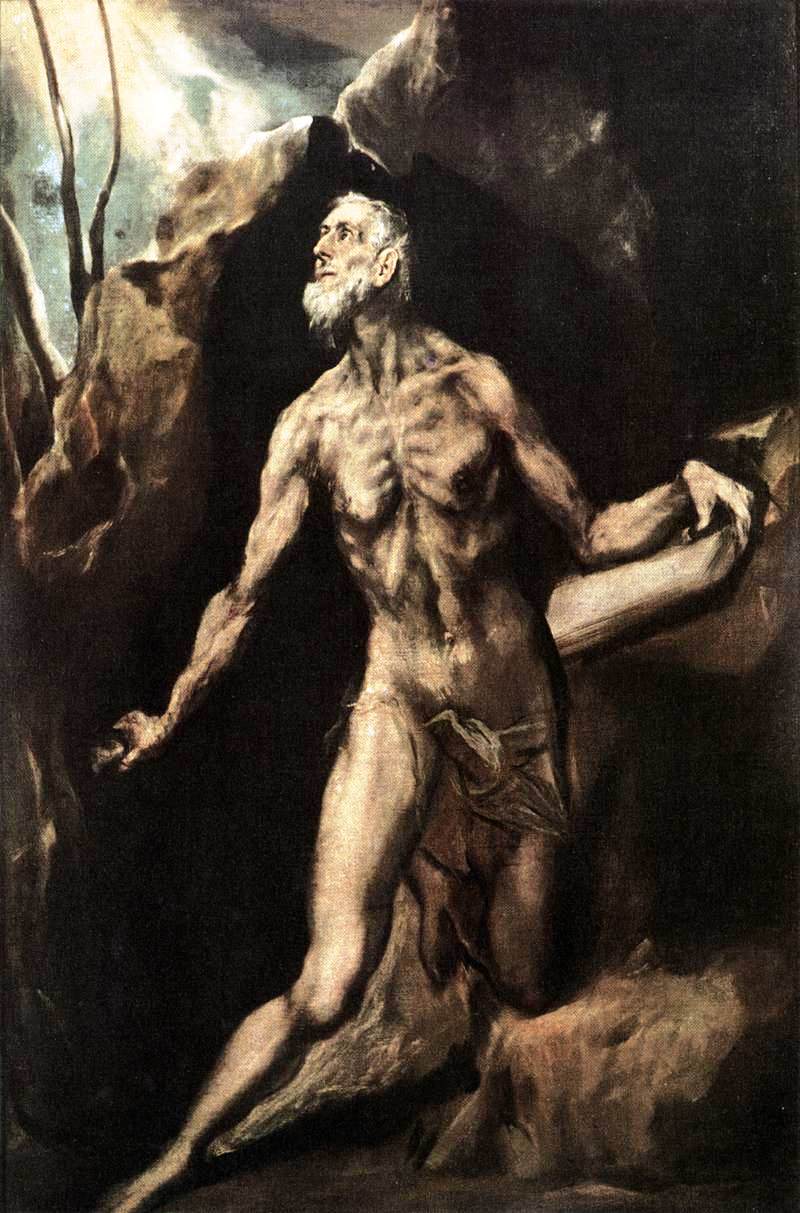The painting is a highly detailed, professional piece of artwork rendered with a range of neutral colors, including black, white, various shades of brown, grey, peach, and blue. It portrays an old, gaunt man in rags, wearing only a tattered loincloth, emerging from or climbing alongside a cave or rock face. His frail body reveals visible ribs and muscles, emphasizing his emaciated state. He has white hair and a beard, and his eyes are directed upward, gazing toward a soft white and yellow light that shines through an overcast sky in the top left corner of the painting. There appears to be a tree in the vicinity of the light. The background behind him transitions from the dark depths of the cave to a greyish blue and white sky, adding depth and contrast to the scene. The man seems to be holding onto the rock face with both hands, with one knee bent on a smaller rock and the other leg stretched out, indicative of climbing or emerging from the cave. The thoughtful use of color, lighting, and detailed anatomy adds to the provocative and dark nature of the artwork.